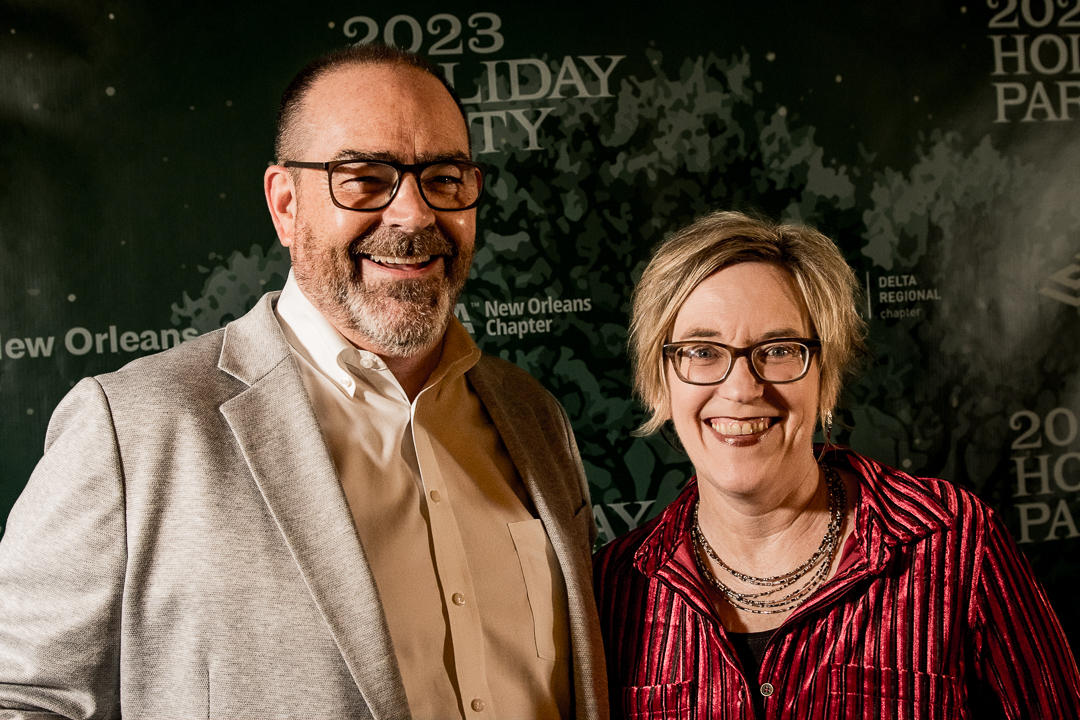In this horizontally aligned rectangular image, a close-up captures a man on the left and a woman on the right, both smiling directly at the camera. The background features a black and gray wall with the text "2023 Holiday Party" in gray, and smaller text reading "New Orleans Chapter" along with "Delta Regional." The man, appearing older, sports a gray suit jacket over a tan collared button-down shirt and wears brown, rectangular glasses. His hair is shaved very short, revealing a balding top with gray sides that match his short facial hair. To his right, the woman, wearing black rectangular glasses, radiates a big smile accentuated by deep red lipstick. Her short blonde hair falls just past her ears. She dons a vertically striped shirt in red and black, complemented by several black or silver chains around her neck. They appear to be the central focus of this indoor setting, possibly at an event based on the background text.